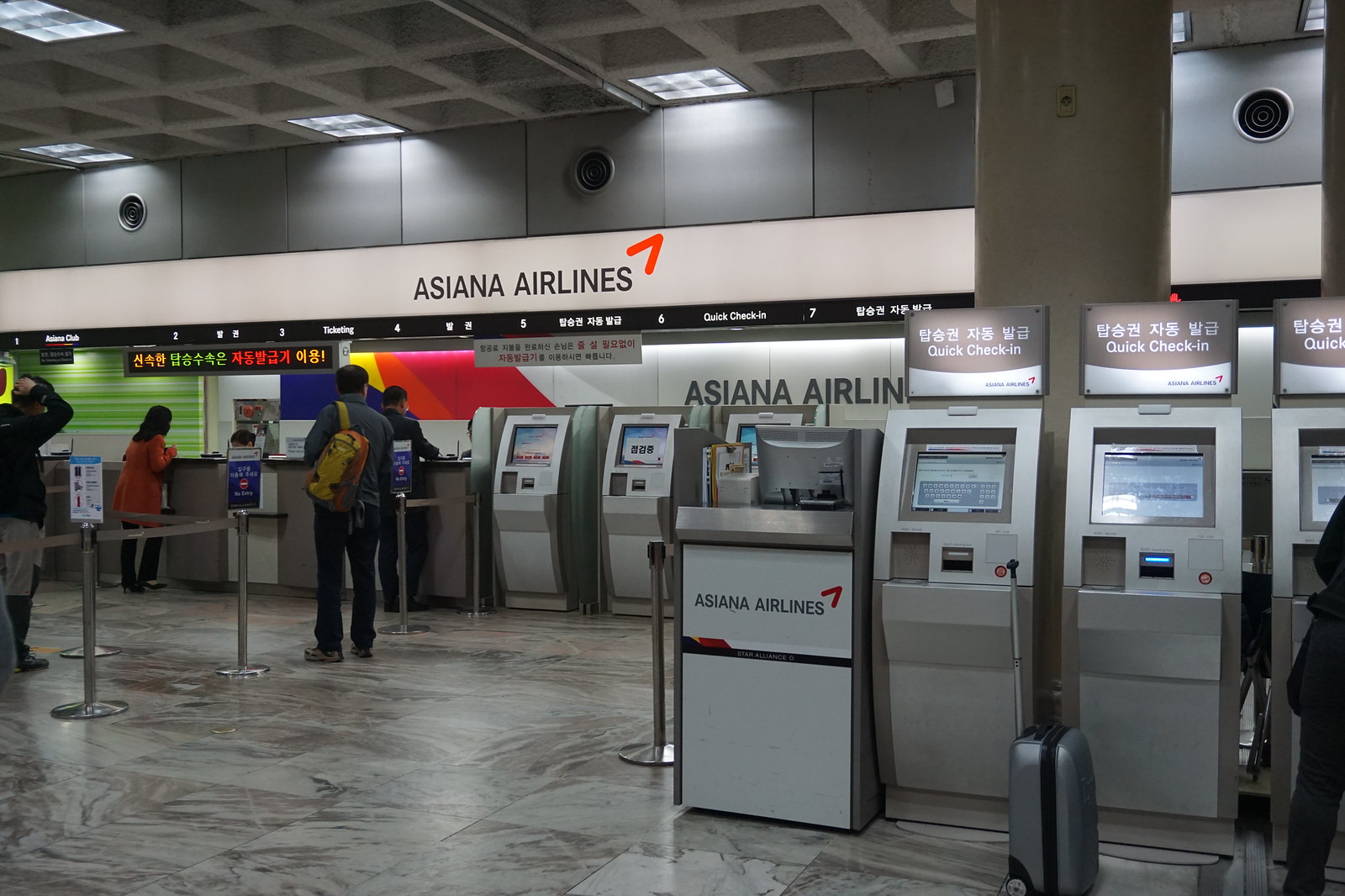This photograph captures the bustling check-in area of an airport, specifically for Asiana Airlines. On the right side, a series of self check-in kiosks are lined up beneath a sign that reads "Quick Check-In." A person stands partially outside the frame at the far-right kiosk. In contrast, the left side features a more traditional check-in setup with rows of people lined up, guided by leather rope straps, waiting for assistance from human attendants. Above these rows, signs bearing the Asiana Airlines logo and a distinctive red arrow are prominently displayed. The floor is covered with gray square tiles, and the backdrops behind the check-in desks are vividly colorful, featuring green stripes and bold sections of blue, yellow, red, and white. The ceiling lights, set into a sleek, grayish-silver toned ceiling, cast a functional glow over the scene, adding to the typical airport ambiance.